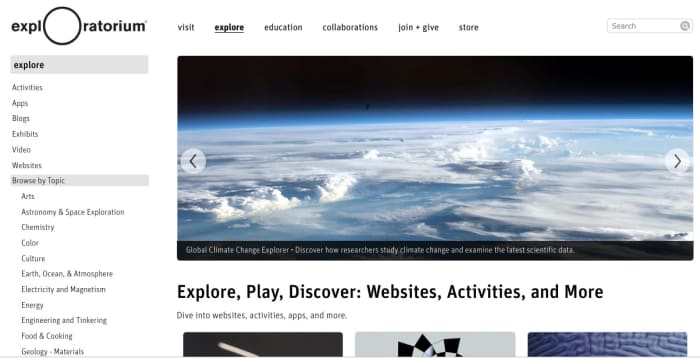The image depicts a detailed webpage from the Exploratorium website. The top left corner features the word "Exploratorium," creatively stylized with "E-X-P-L," a large circular 'O,' followed by "R-A-T-O-R-I-U-M." Directly to the right, the navigation menu includes the options: Visit, Explore, Education, Collaborations, Join & Give, and Store, with "Explore" prominently highlighted in bold and underlined. Adjacent to these options, on the far right, is a search bar.

On the left side of the webpage, a vertical menu lists: Explore, Activities, Apps, Blogs, Exhibits, Videos, Websites, or Browse by Topic. The topics available for browsing include Arts, Astronomy and Space Exploration, Chemistry, Color, Culture, Earth, Ocean and Atmosphere, Electricity and Magnetism, Energy, Engineering and Tinkering, Food and Cooking, and Geological Materials.

The main content on the right side of the image features a striking photograph taken from space, showcasing the Earth’s surface and clouds. Below this image is the title "Global Climate Change Explorer," accompanied by a subtitle: "Discover how researchers study climate change and examine the latest scientific data." Further down, bold black text invites users to "Explore, Play, Discover Websites, Activities, and More," followed by a call-to-action in a less bold font: "Dive into Websites, Activities, Apps, and More."

The overall layout is designed to engage users with a blend of visuals and text, emphasizing the exploration of various scientific and educational topics.